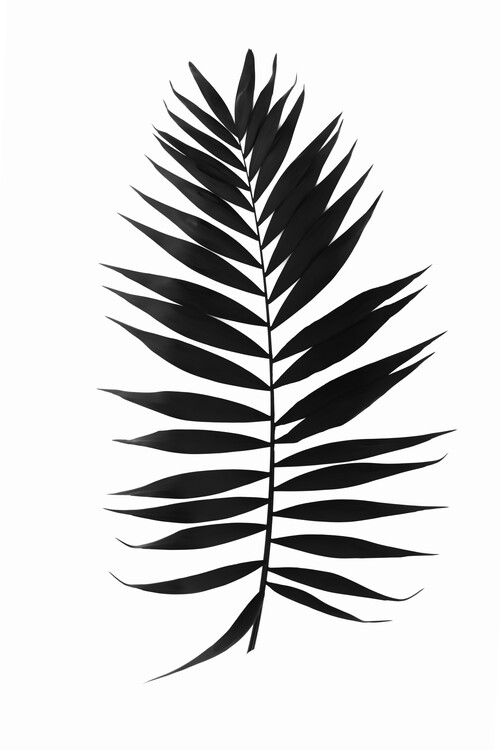This image features a digitally-created, black and white depiction of a long stem with multiple leaves branching from it, set against an off-white background. The slender stem, which appears to be black, rises from the bottom center of the image and slightly curves to the left. Along the stem, pairs of small, thin leaves emerge symmetrically on both the left and right sides, widening in the middle and tapering at the tips. At the top, two larger leaves extend upwards, one angling to the left and the other to the right. A thicker leaf also projects downwards from the base of the stem. The composition is balanced and occupies most of the image space, emphasizing the central positioning of the object with no additional text or elements, giving it a clean and focused look suitable for digital presentations or graphic design uses.